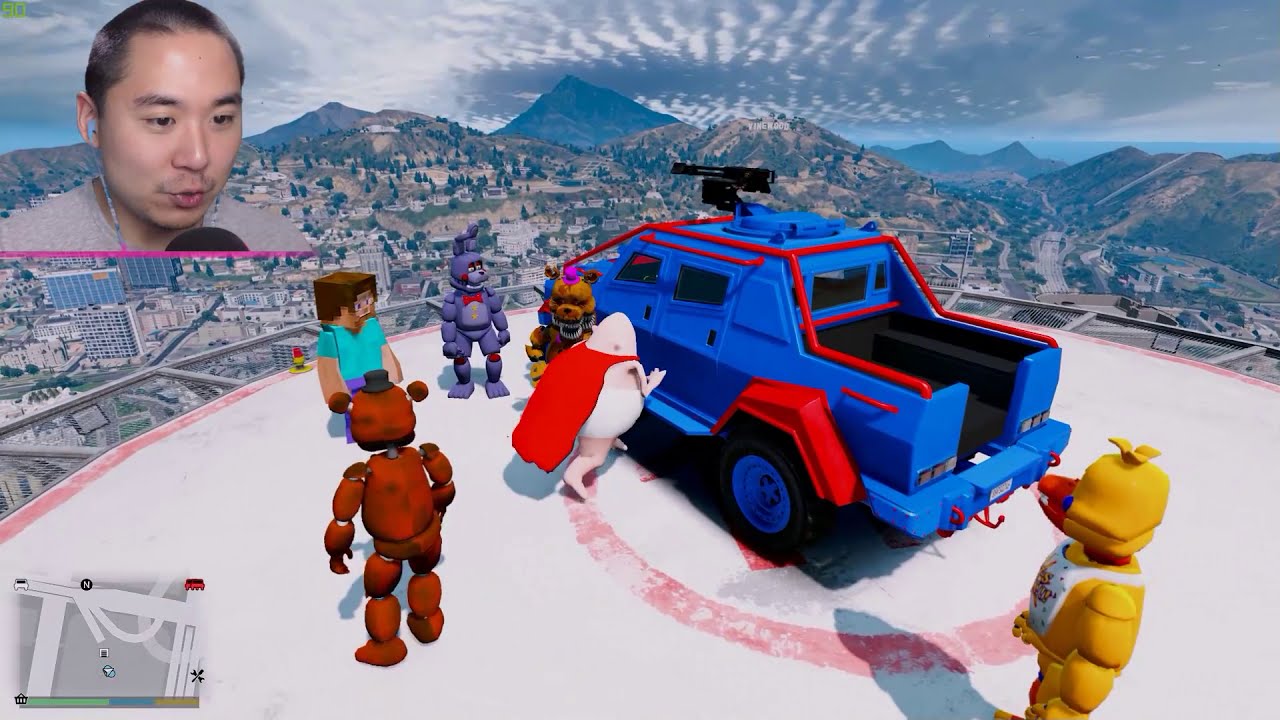In this detailed rectangular image, approximately three inches tall by six inches wide, we observe a streamer, an Asian male with very short hair and black eyebrows, speaking into a visible microphone in the upper left-hand corner. The background behind him is transparent, allowing us to see the vibrant video game he is playing. Dominating the center of the screen is a circular white platform, elevated high above a sprawling cityscape with highways, mountains, and a sky dotted with clouds.

Prominently situated in the middle of this platform is a blue Jeep with red accents, featuring a black gun mounted on its roof. This vehicle is nearly centered in the image. Surrounding the Jeep are familiar characters such as Steve from Minecraft, multiple animatronic figures from Five Nights at Freddy's (including a yellow duck), and Captain Underpants, who appears to be preparing to enter the vehicle.

In the lower left-hand corner of the image, there is a small square showing the map of this video game setting. The ledge and its vivid details - with colors spanning white, grey, green, blue, light blue, yellow, red, and orange - suggest a dynamic and animated game environment. Overall, the scene conveys an engaging moment captured from a streamer's live gameplay session, filled with colorful characters and an impressive aerial view of the game's extensive landscape.